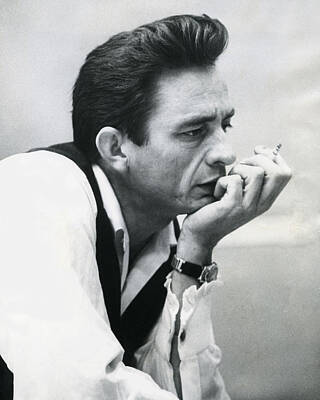This is a black and white side-view photo of Johnny Cash, capturing him in a pensive, contemplative moment. He rests his chin in his hand, with his fingers curled around a cigarette. Johnny is styled in a white collared shirt with a black vest, and the cuff of his visible sleeve is unbuttoned, giving him a slightly disheveled appearance. He wears a watch with a black band and a silver clasp. His hair, reminiscent of a 1950s pompadour, is thick, full, and slicked back, standing about an inch above his forehead before sweeping backwards. With furrowed eyebrows, he gazes pensively, almost solemnly, into the distance. The backdrop is a light gray, setting off the striking contrast of the black and white image.